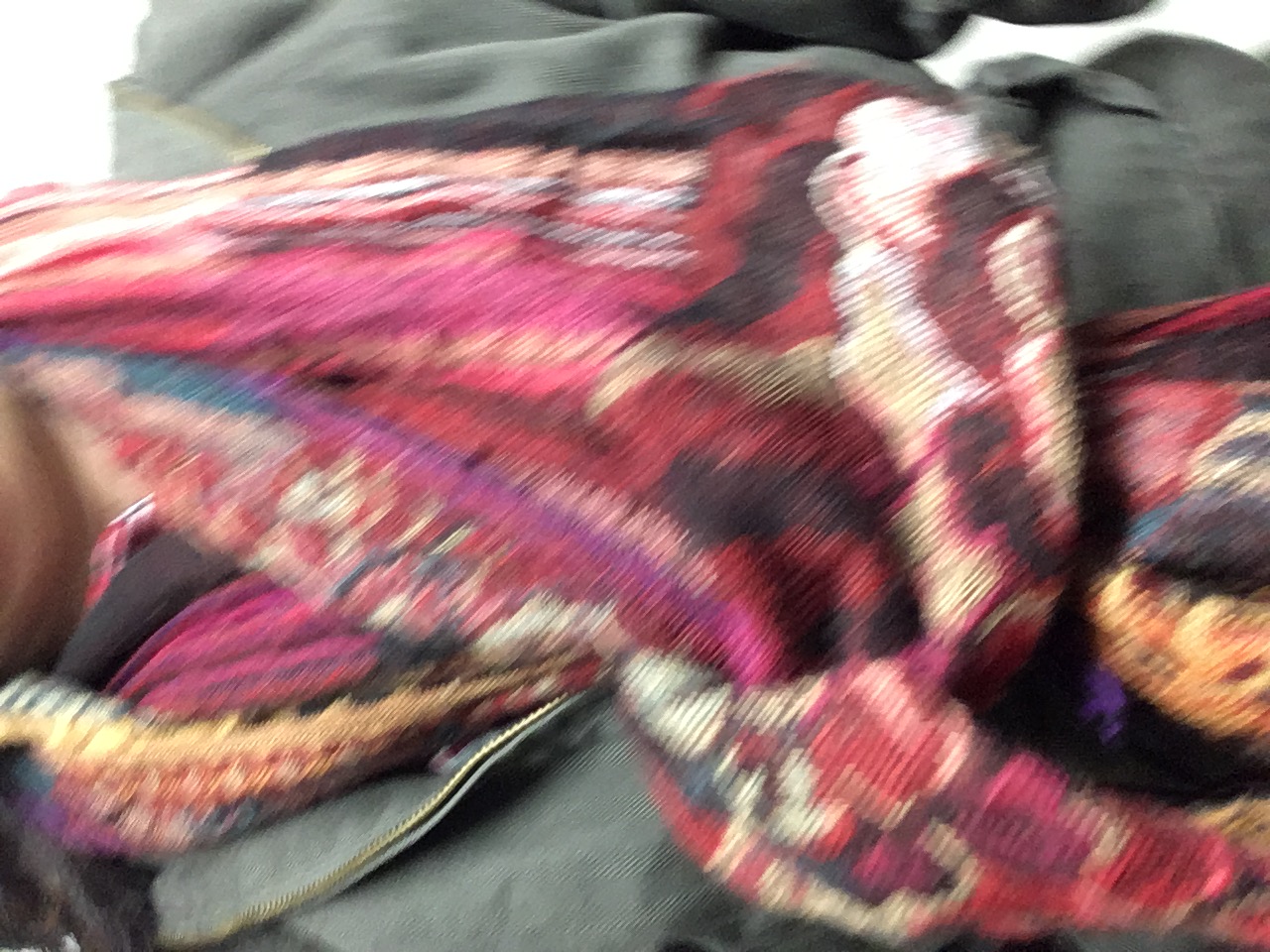The image depicts a slightly blurry person positioned in front of the camera lens, captured from the neck down to the waist, though no arms are visible. The individual is dressed in a grey jacket adorned with gold zippers, despite one description referring to the jacket as green. A vibrant, multi-colored scarf wraps around the neck and drapes down the front of the jacket, displaying an array of hues including purple, pink, orange, yellow, red, and beige. The scarf, featuring possibly indistinct squiggly lines or an elaborate floral design, adds a rich textural contrast to the subdued jacket. There is a noticeable light glare in the upper right-hand corner of the image, further contributing to the overall blurry and bright ambiance.